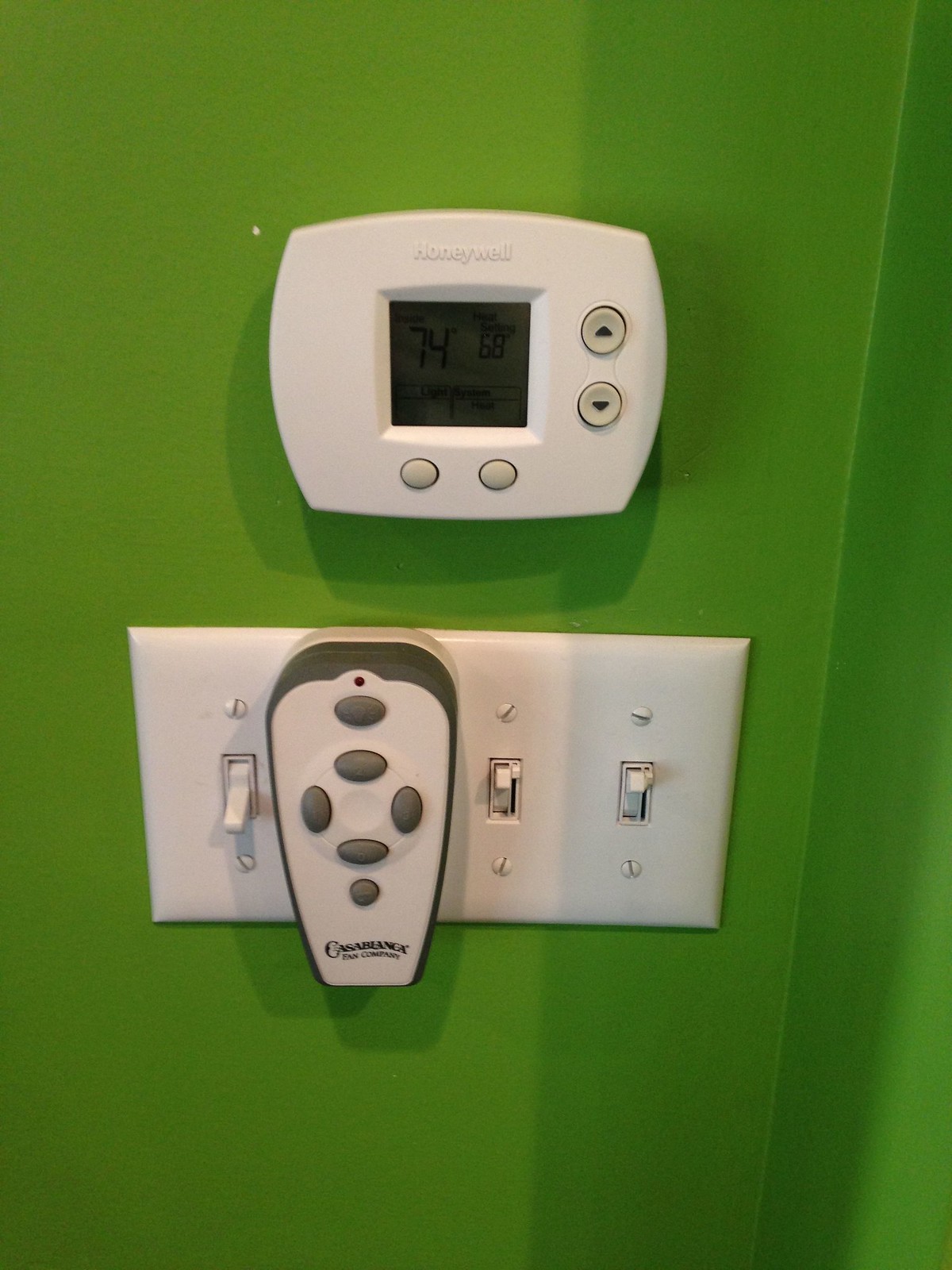The image features a bright, pea-green wall with varying shades, prominently displaying a white Honeywell thermostat. This thermostat includes a digital display that shows the current temperature, with the numbers "74" and "68". On its right side are two gray buttons with black arrows for temperature adjustment—an upward pointing arrow on the top button and a downward pointing arrow on the bottom button. Beneath the display are two additional round buttons. Directly below the thermostat is a white light switch panel with four switches, the first switch facing down (off), and the third and fourth switches facing up (on). The second switch spot is occupied by a remote control for a Casablanca Fan Company. This remote has a gray exterior with six buttons—five oval-shaped and one circular—displaying the company’s name in black.